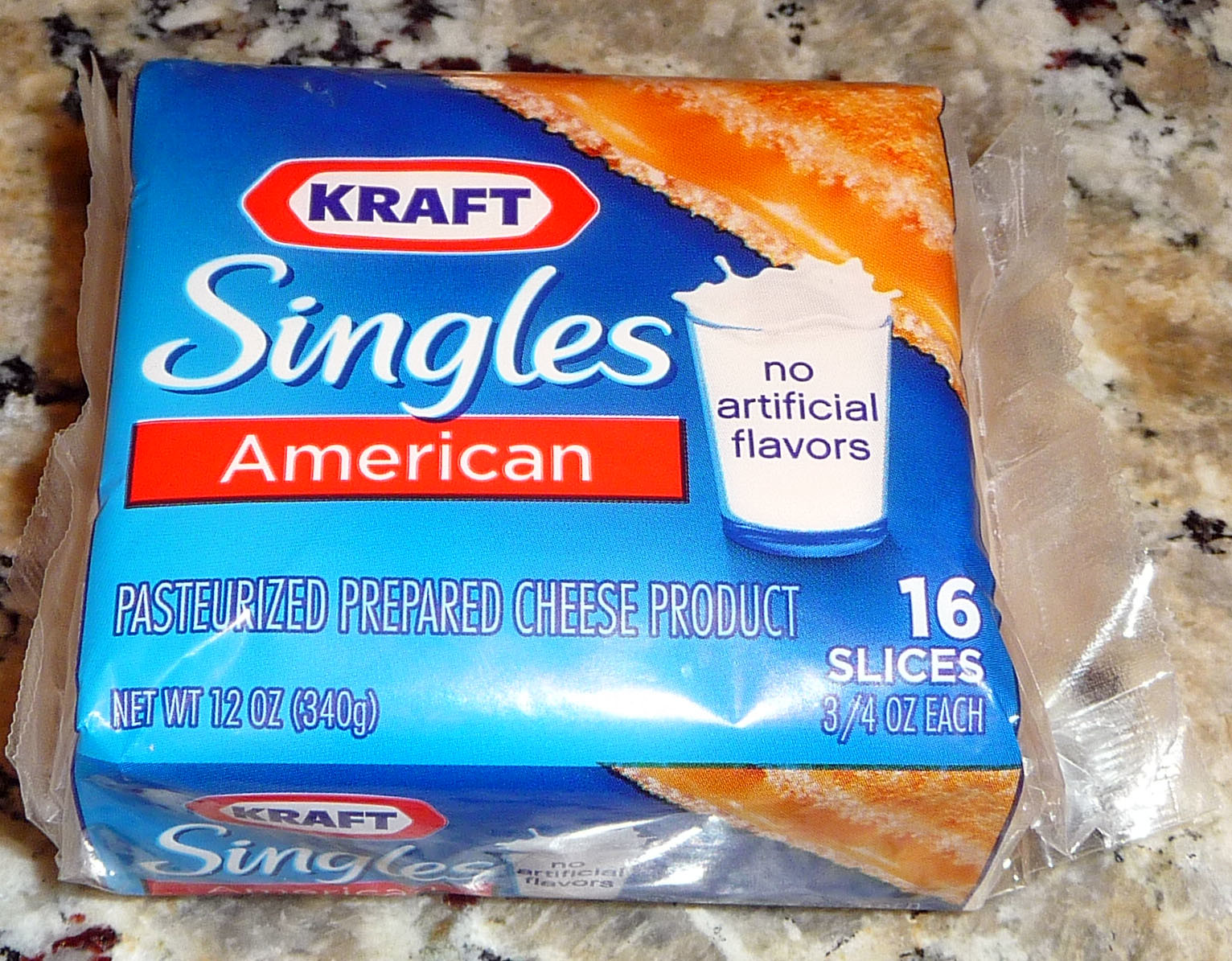A detailed close-up photograph showcases a package of Kraft Singles American cheese. The cheese is wrapped in its iconic plastic packaging, prominently displaying the "Kraft Singles American" label. An illustrated glass of milk, shown with milk splashing out, is depicted on the package, accentuated by the statement "No Artificial Flavors." Just below this illustration, the text "Pasteurized Prepared Cheese Product" is clearly visible. At the bottom right corner of the package, the label indicates that it contains "16 Slices." The photograph, taken with a flash or a bright light source, highlights the shiny plastic wrapping, creating noticeable highlights and reflections.

The package appears to be unopened, with the plastic wrapping intact and slightly protruding from the left and right sides. The bottom of the package is folded under, revealing a glimpse of the front and side labels. The vibrant colors of the packaging—orange, white, blue, red, and light blue—stand out against the granite countertop on which it rests. The countertop features a mix of brown, black, and gray hues, providing a contrast to the bright packaging of the cheese.